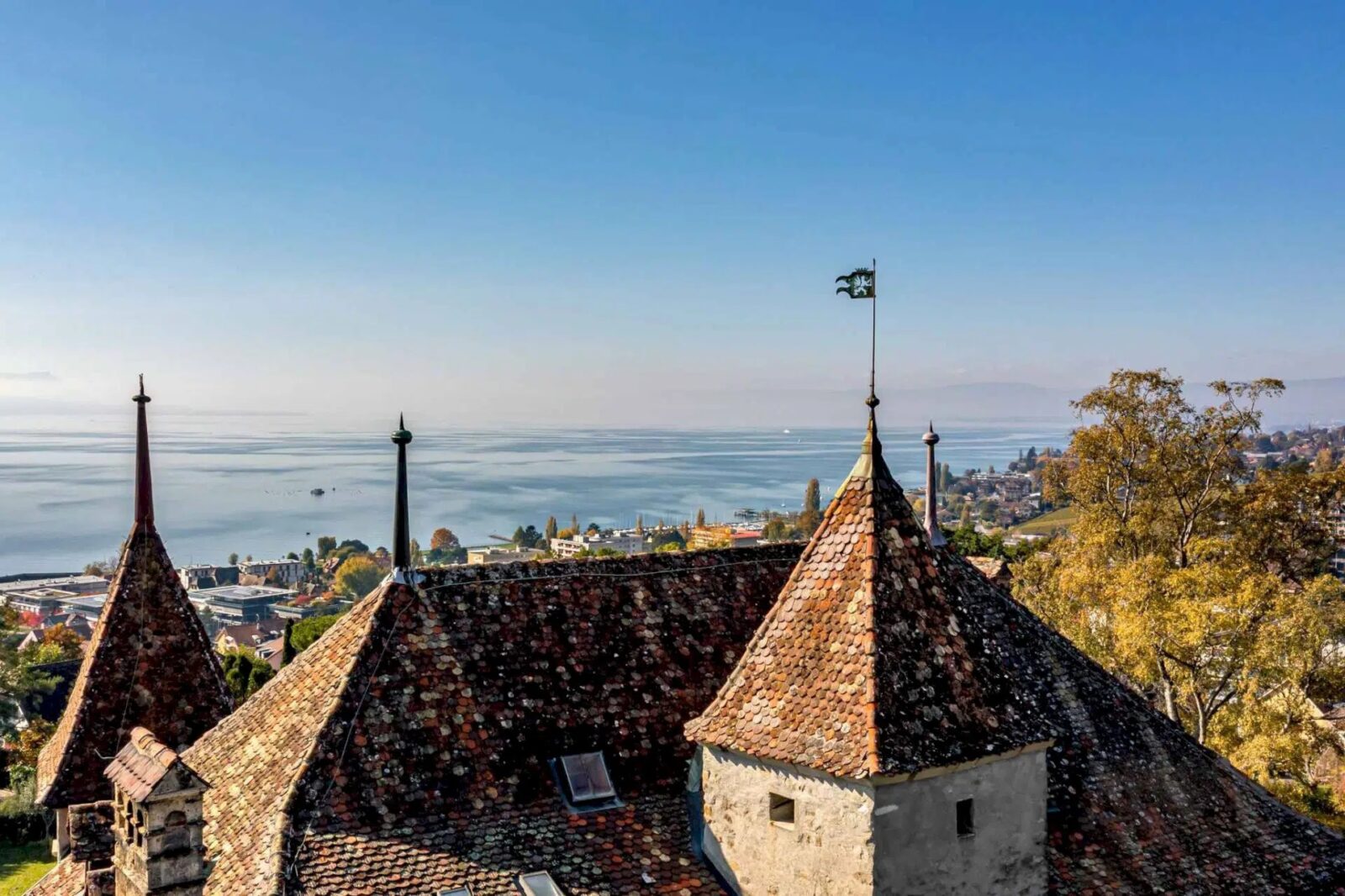The image depicts a picturesque seaside cityscape taken from an elevated vantage point. In the foreground, numerous rooftops dominate the view, including prominent buildings with pointed, pyramidal spires adorned with small flags. These structures are accompanied by regular-sized city buildings, creating a dense urban texture. To the right, a cluster of trees adds a touch of greenery to the scene. Stretching into the distance, the expansive ocean forms a stunning backdrop, with the coastline extending from the left to the right of the frame. Above, the sky is a clear, bright blue, enhancing the overall clarity and luminosity of the daytime setting. The muted color palette features shades of brown, off-white, blue, and subtle green tones, suggesting a tranquil and perhaps slightly vintage atmosphere. While the image feels realistically detailed, hints of blurriness raise the possibility that it might be a digital rendering or a scene from a video game.